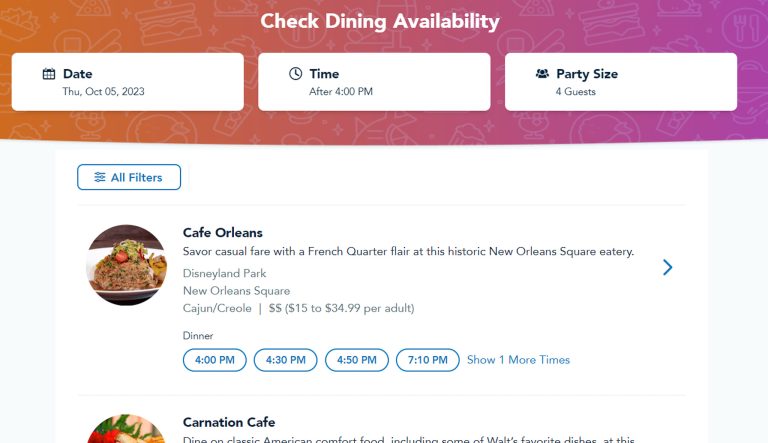**Caption:**

This image is a screenshot of a desktop application showing dining availability search results. The user interface features a stylized banner gradienting from orange to hot pink, displaying various food items and plates. Below the banner, three horizontal boxes show search parameters: Date set to Thursday, October 5th, 2023; Time after 4 PM; and Party Size for 4 guests. 

Underneath these parameters is a white box with a blue label on the top left corner reading "All Filters." Below this label is a thin gray line. 

The first dining result showcases an image of a white plate filled with a rice dish from "Cafe Orleans." The description reads: "Savor casual fare with a French Quarter flair at this historic New Orleans Square eatery." This establishment is located in Disneyland Park, specifically in New Orleans Square, offering Cajun/Creole cuisine. The price range is indicated as $$ with the note, "$15 to $34.99 per adult." Available dinner times are 4:00 PM, 4:30 PM, 4:50 PM, and 7:10 PM, with an option to "Show one more time." A small forward arrow is located in the top-right corner of this result entry.

The second result, partially visible below, features "Carnation Cafe." It describes the offering of classic American comfort food, including some of Walt Disney's favorite dishes, though the text gets cut off and the full description is not visible.